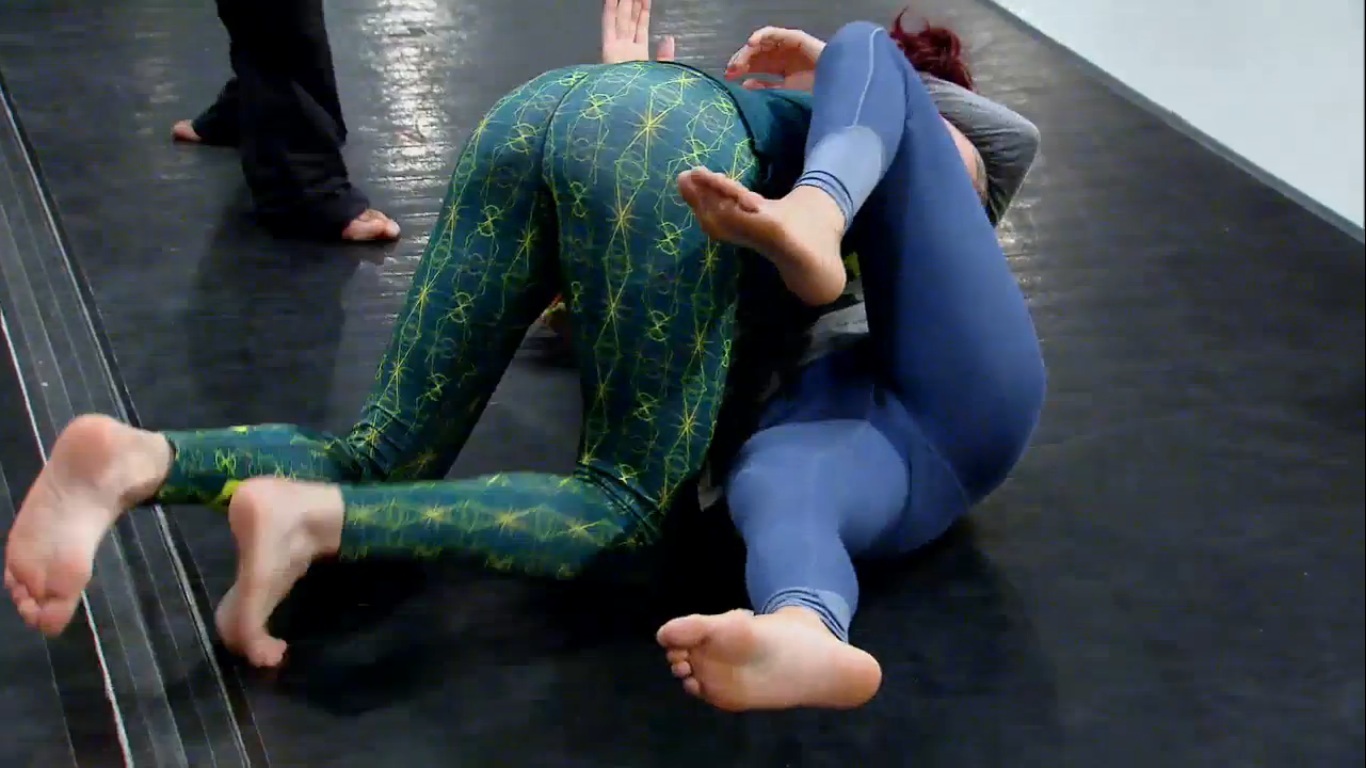In this image, the scene is set on a black mat positioned against an off-white wall that runs along the left and right sides. On the left, a person is captured mid-movement, stepping forward with their bare foot and clad in long black pants. They seem poised and ready for action, with their other foot positioned directly behind them. A grey, double line is visible on the left side of the mat, possibly marking an area or boundary.

Two barefooted combatants, who appear to be female, are central to the scene. The first combatant on the left is dressed in vibrant green tights adorned with yellow lines and diamond patterns that run along their legs. They are wearing a dark green top and have reddish hair, adding to their striking appearance. Appearing to be in motion, they hover over the second combatant, who is lying down on the mat.

The second combatant is dressed in tight-fitting blue pants and a grey top. With their hands raised, poised to either defend or counter, they are directly beneath the first combatant. This dynamic moment captures the tension and readiness in their postures, with the first combatant seemingly about to engage with the second.